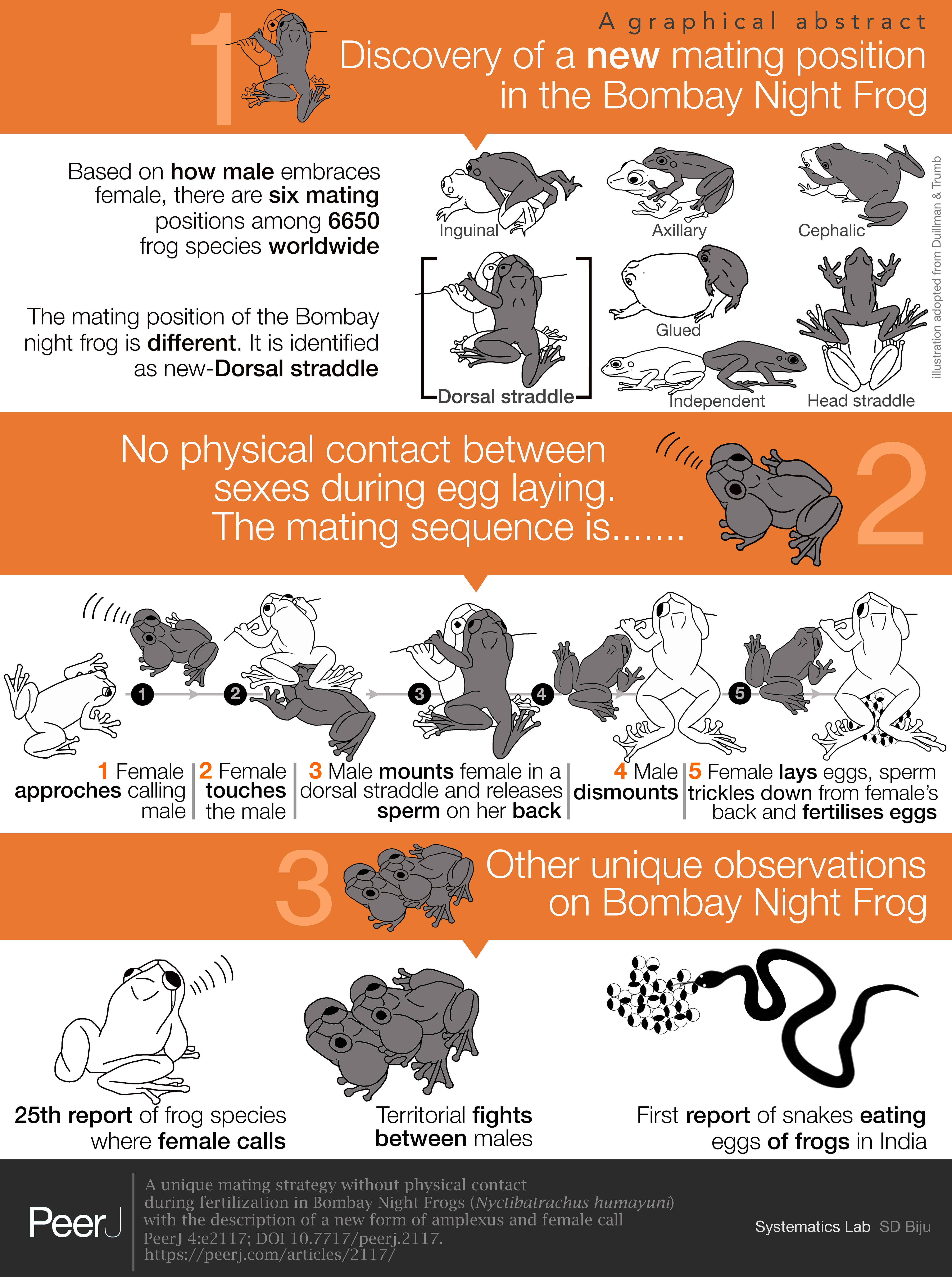The image is a detailed informational chart, primarily alternating between orange and white sections, providing a graphical abstract titled "Discovery of a New Mating Position in the Bombay Night Frog" in gray font at the top. The top orange banner introduces this theme, followed by illustrations of mating frogs—one white and one dark gray. To the left of these illustrations, black text explains that there are six mating positions among 6,650 frog species worldwide, with the Bombay Night Frog having a unique "new dorsal straddle" position.

Below, another orange banner in white font reads: "No physical contact between sexes during egg laying." The subsequent white section details the step-by-step mating sequence through illustrations: (1) Female approaches, calling male; (2) Female touches male; (3) Male mounts female in a dorsal straddle and releases sperm on her back; (4) Male dismounts; (5) Female lays eggs as sperm trickles down from her back, fertilizing the eggs.

The final part, marked by another orange banner and white font, is titled "Other Unique Observations on Bombay Night Frog." A white section underneath lists these observations, mentioning the 25th report of a frog species where the female calls, territorial fights between males, and the first report of snakes eating frog eggs in India. The chart uses a mix of dark gray, black, white, orange, and off-white colors and appears to be digitally created.